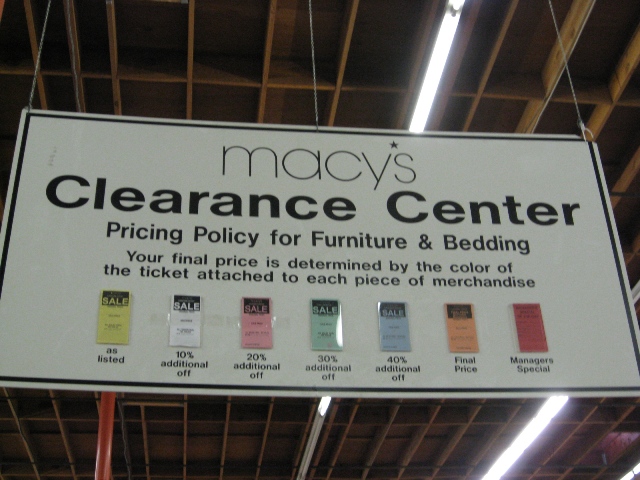This photograph depicts the interior of a department store, specifically Macy's Clearance Center. The ceiling is characterized by exposed wooden rafters and fluorescent lights that run from the forefront towards the back of the image.

Centrally positioned and suspended from the ceiling by metal wires is a large, white sign with black trim. The top of the sign features the text "Macy's Clearance Center" in bold black letters. Below this heading is a detailed description of various discounts available at the store.

Towards the bottom of the sign, seven smaller sale signs are displayed, each in a different color: yellow, white, pink, green, blue, orange, and red. Each of these smaller signs lists specific discount amounts. For example, the yellow sign on the far left reads "As Listed," while the remaining signs contain other discount details, offering a visual guide to the various savings available throughout the store.